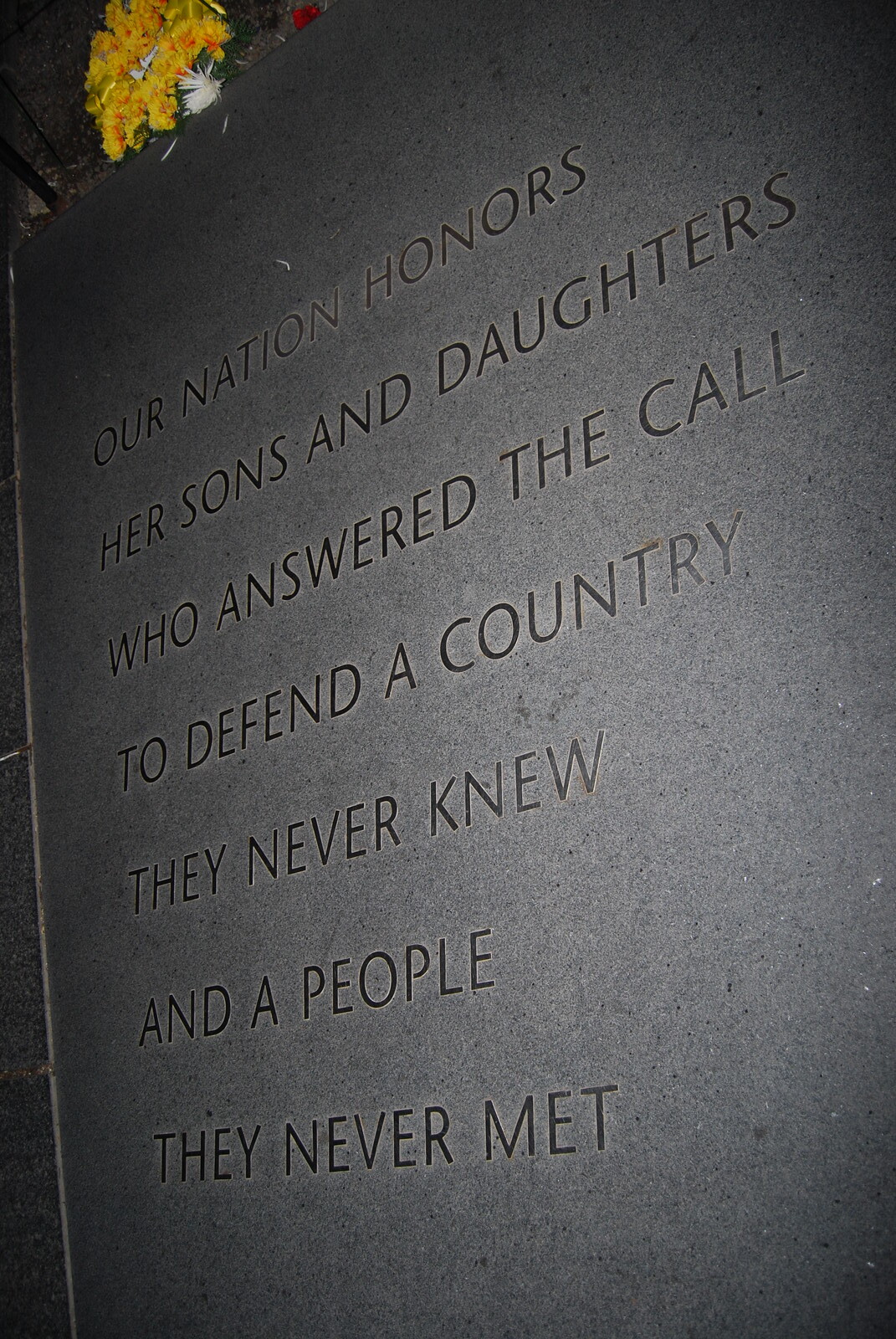The image shows a dimly lit, dark gray metal plaque mounted against a cement surface, viewed from an angle. Illuminated by the night, the engraving reads: "Our nation honors her sons and daughters who answered the call to defend a country they never knew and a people they never met." Atop the plaque is a small bouquet of yellow flowers, adding a poignant touch to the solemn tribute. There are no other noticeable objects, and the image is clear in its depiction despite the low lighting.